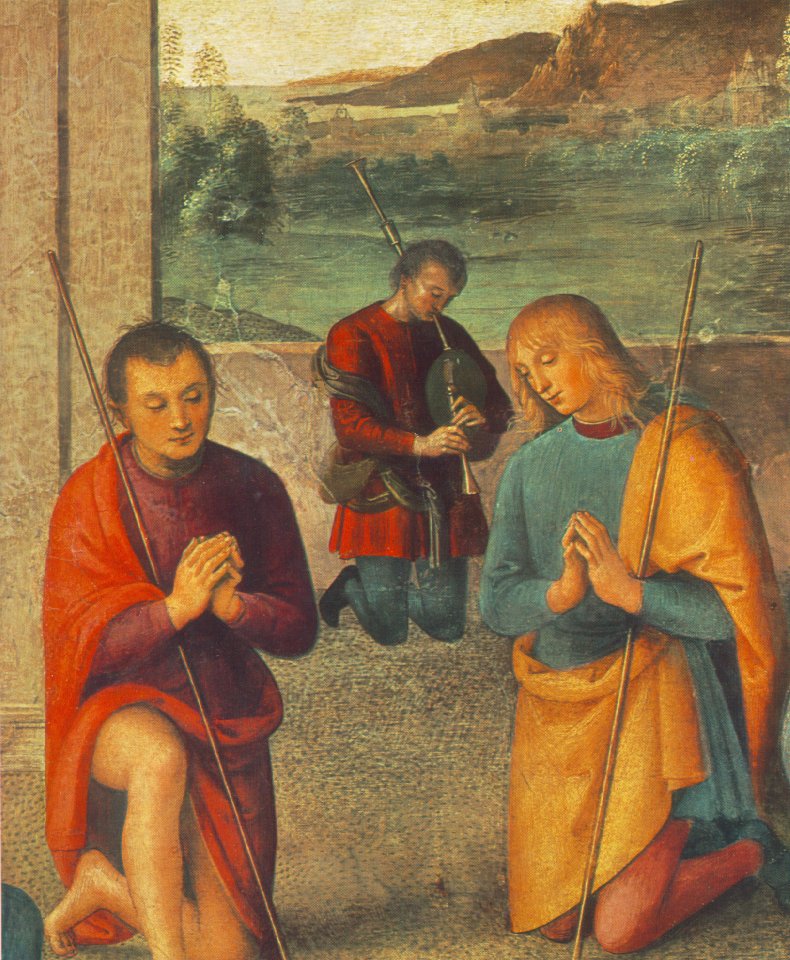This detailed painting depicts an outdoor scene with three individuals kneeling in prayer at the center. The person on the left is wearing a red robe paired with a purple shirt, and he is kneeling on his right knee while his left knee is bent. This figure has short black hair and holds a staff in the crook of his right arm. Adjacent to him, the second person is kneeling on both knees, dressed in light blue and yellow, and has long blonde hair; his hands are clasped together in prayer. The third figure, further back, is also kneeling on both knees. This individual is adorned in a red tunic and blue pants and appears to be playing an instrument, likely a flute. All three figures have staffs leaning against their bodies.

The backdrop of this scene features a serene body of water, mountain ranges with an orange hue, and a sky that mixes white and tan shades. There are trees scattered both in the distance and up close on a land formation. The painting's color palette includes browns, reds, tans, blues, greens, oranges, yellows, and golds, suggesting a harmonious balance between foreground and background elements. The scene evokes a historical atmosphere, possibly from the 12th century, and the style seems fitting for display in an art show or museum.